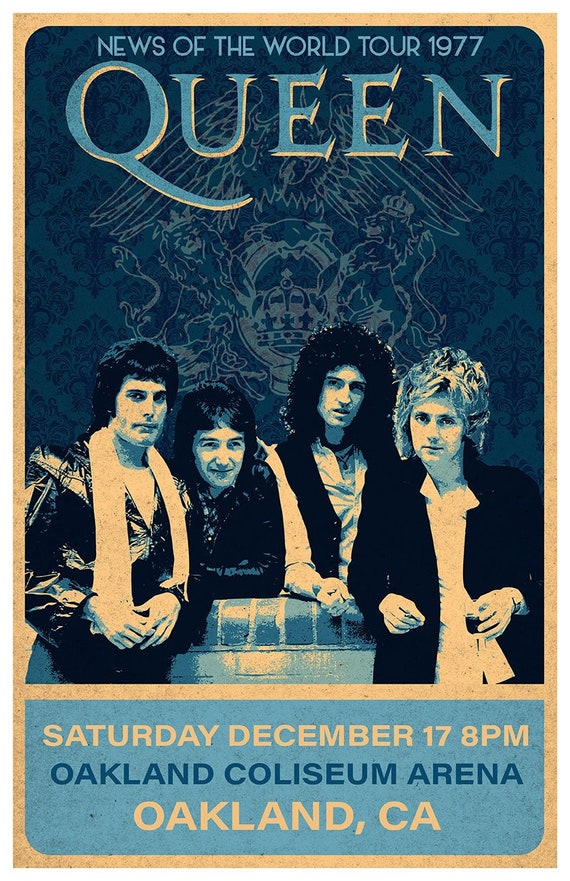This vintage concert poster for Queen's "News of the World Tour 1977" prominently features the band's name in a blue font with a slightly white outline at the very top. Below this, the four band members are lined up and looking towards the viewer. On the far left, a man with medium-length hair is wearing a white scarf and a leather jacket. Next to him, another man with similar dark, medium-length hair also sports a leather jacket. To the right, a member with very long, curly black hair wears a white long-sleeve shirt that appears to be a vest. The farthest right band member has long, lighter-colored hair and is dressed in a light-colored undershirt with a collar and a black jacket. The event details are listed beneath the band members: in slightly aged white text, it reads "Saturday, December 17, 8 p.m." followed by "Oakland Coliseum Arena" in blue, and "Oakland, California" again in white. The overall background of the poster features graphic elements, predominantly in blue, and a faded tan edge around the perimeter. The background also includes a partially visible logo or graphic that enhances its aged, nostalgic feel.